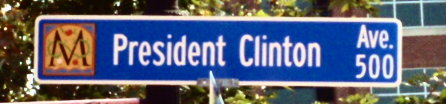A detailed close-up image showcases a blue street sign with a white border and white text reading "President Clinton". The sign is rectangular, and the image is tightly cropped to focus solely on the sign. Additionally, the sign displays "EV 500" on the side. To the left, there's an intriguing square design featuring blue corners at the top and a fully blue bottom. This design encompasses a large black letter "N", entwined with a green vine-like graphic that appears to have fruits, though the details are blurry. The background comprises lush green trees and leaves, adding a natural contrast. On the right side of the image, part of a brick building facade with windows is visible, possibly hinting at a school or institutional structure.